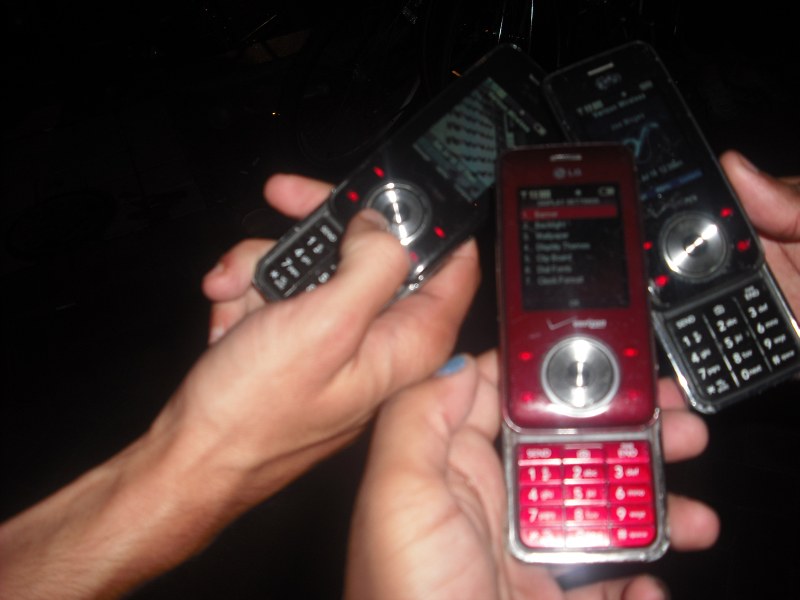In this blurry nighttime photograph, three hands with light skin tones, likely belonging to two males and one female with blue nail polish on her thumb, hold vintage LG slide Verizon phones. The scene is set against a completely black background, highlighting the retro devices. The central phone is red with a large rectangular screen and a round knob in the middle, seemingly bearing the Verizon logo. The phones on either side are black with gray accents; the left one has a round dial in the center with the thumb resting on top, while the right one features a silver knob surrounded by four red dots. Despite the image's low resolution and hazy quality, it captures a moment of shared nostalgia and showcases these old model phones in varying colors.